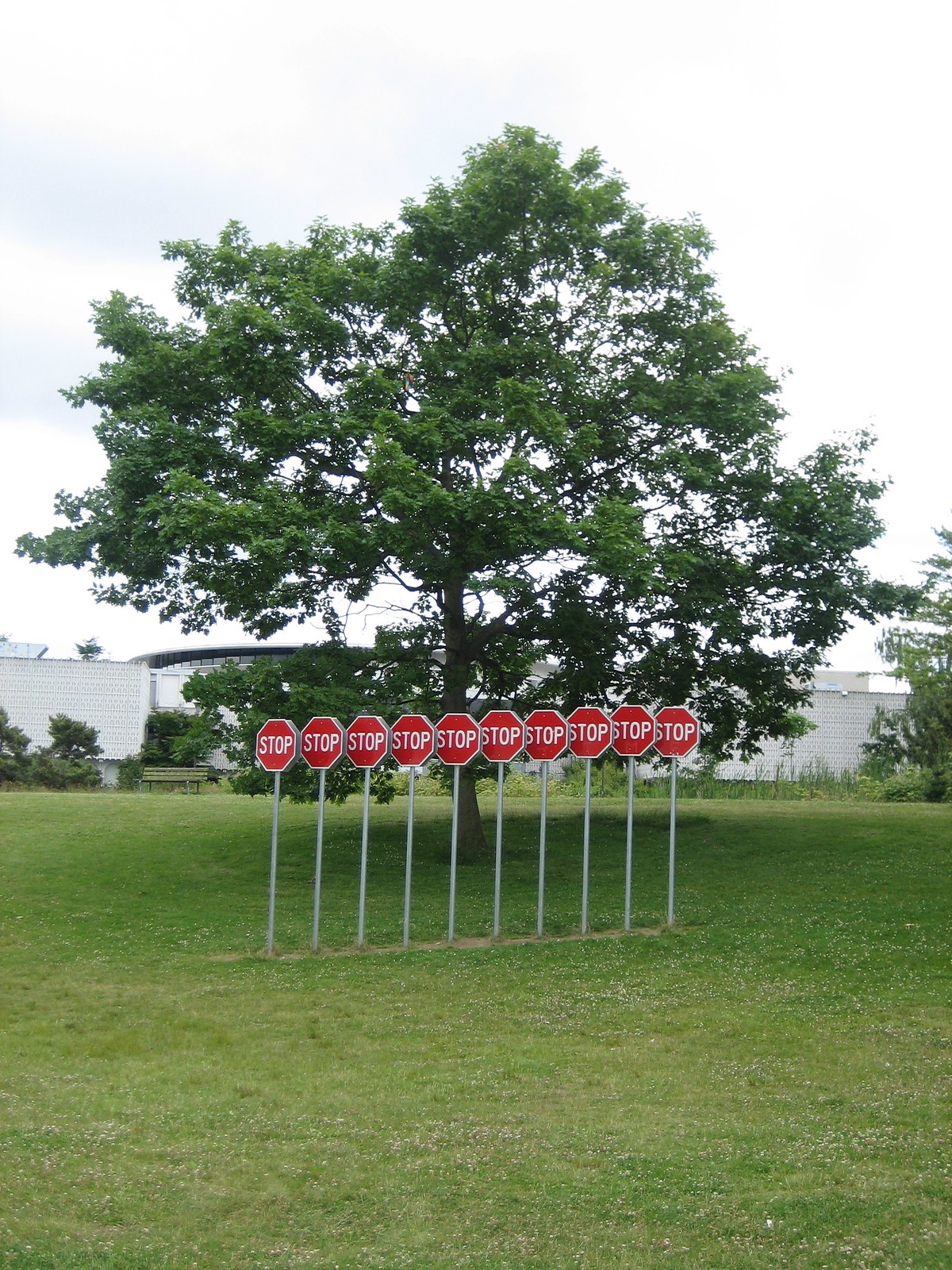This detailed outdoor photograph captures a surreal scene featuring a neatly trimmed, lush green meadow with a prominent solitary tree at the center, surrounded by dense green foliage. In front of the wide, verdant tree, which may be a maple, stand ten evenly spaced stop signs, each mounted on a slender silver pole. These standard hexagonal red signs with white "STOP" text form a curious display, aligned in a precise row. In the background, partially obscured by leafy bushes and shrubs, sits a large white building, adding to the enigmatic composition under a mostly cloudy sky, tinged with faint grayish-blue hues.